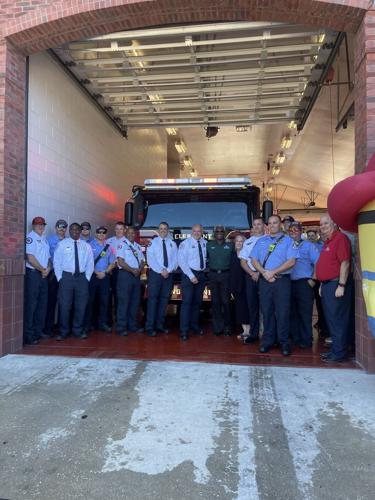This photograph captures a group of men, presumably a team of firefighters, standing in front of a fire truck inside a fire station. They are lined up in a horizontal row beneath a high garage with a bricked arched opening. The station's interior features clean white brick tiled walls and a red tile floor. All the men are uniformly dressed in dark blue trousers, long-sleeved light blue button-down shirts, and black ties, except for one man on the far right sporting a red short-sleeved collared t-shirt, possibly indicating a higher rank or different role. The wet tire tracks on the cement driveway just outside the garage suggest recent rain and the recent arrival of the vehicle. Profiles of their faces and hands, some of which are crossed, are visible, indicating a poised and formal photograph.